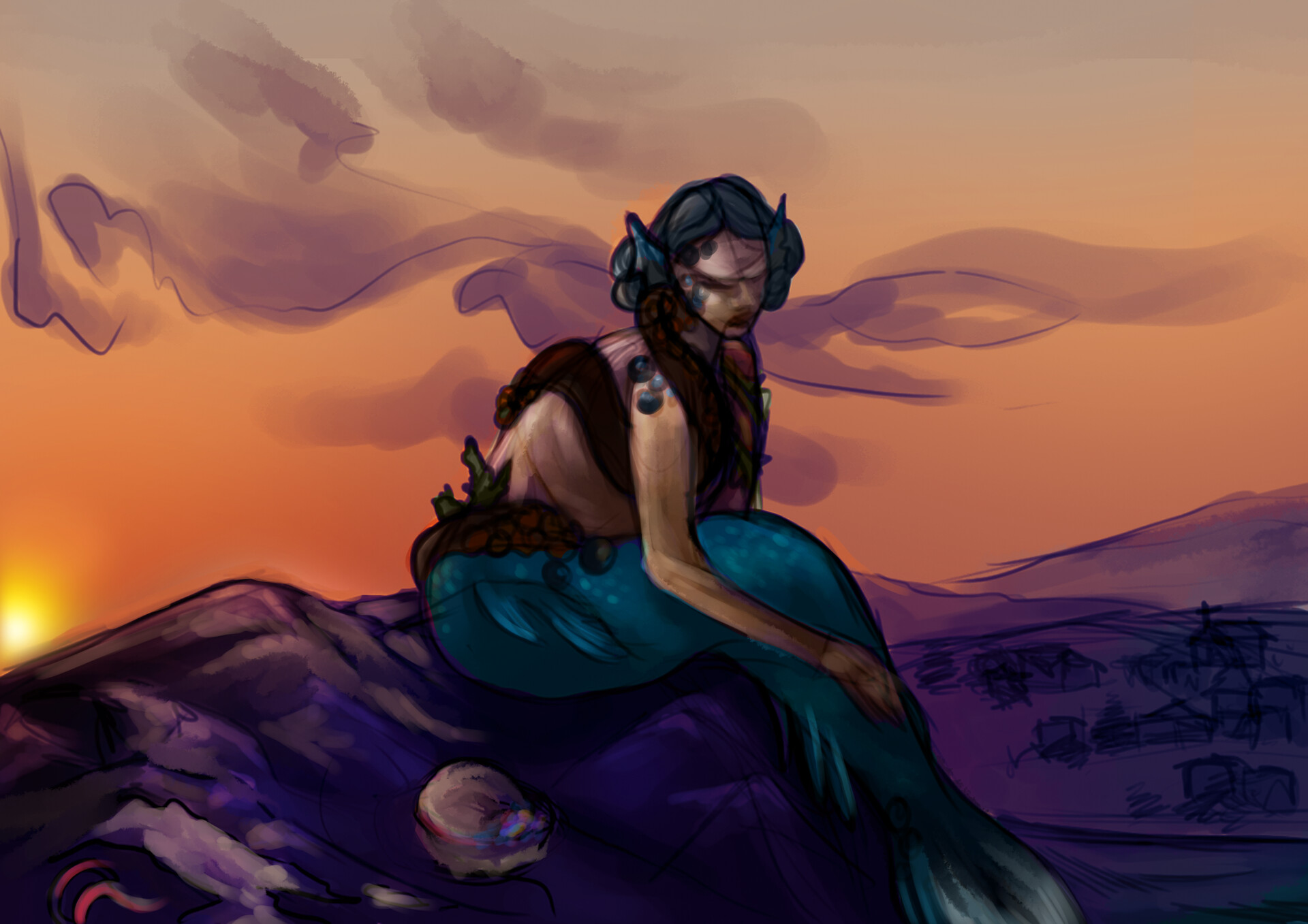The image appears to be a detailed watercolor painting, presenting a contemplative mermaid seated on a purple rock formation. The mermaid, with a blue, scaly tail in place of legs, is hunched over, gazing downward. Her posture is accentuated by one hand resting on her fin, and her bare arm is visible. The mermaid has long, black hair with hints of blue, tied up in buns. She wears a reddish-brown, snake or eel-like garment draped around her torso. The sky forms a striking backdrop with its vibrant orange hue and purple clouds etched with lines. A small, bright yellow sun is situated in the bottom left corner, enhancing the warm tones of the sky. Below these clouds, there are simply drawn buildings, adding an abstract yet whimsical quality to the painting, which predominantly features purple and blue tones. The overall composition, with its emphasis on strong line work and delicate watercolor techniques, gives the piece an unfinished yet intentionally stylized appearance.